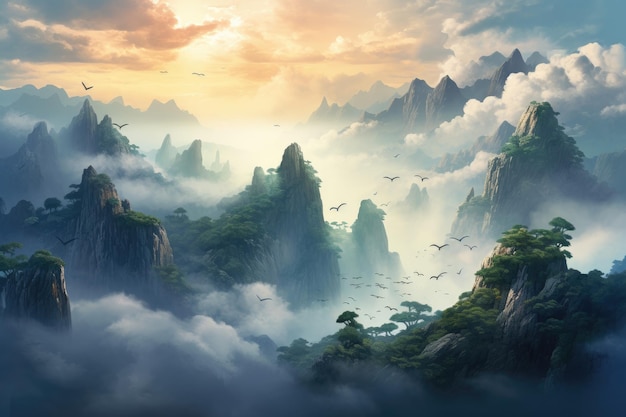This vibrant, AI-generated artwork, styled with a digital painting technique, captures a breathtaking fantasy landscape. Dominated by white, fluffy clouds that blanket the scene, the image showcases numerous lush, green mountaintops piercing through the mist. These steep, jungle-esque cliffs are adorned with leafy trees and frequented by graceful, flying birds. The dramatic cloud cover transitions into a sky tinged with golden-orange hues from a setting sun in the upper left corner. The clouds and misty atmosphere create a mystical ambiance, reminiscent of wuxia or shanxia themes found in Chinese martial arts fantasies. The composition features multiple mountain peaks rising from the clouds, creating a winding valley that guides the eye naturally from the bottom left, through the middle, and to the right, before returning back to the left. The blending of cooler tones in the foreground with the warm glow of the sunset enhances the enchanting and otherworldly feel of this vivid artwork.